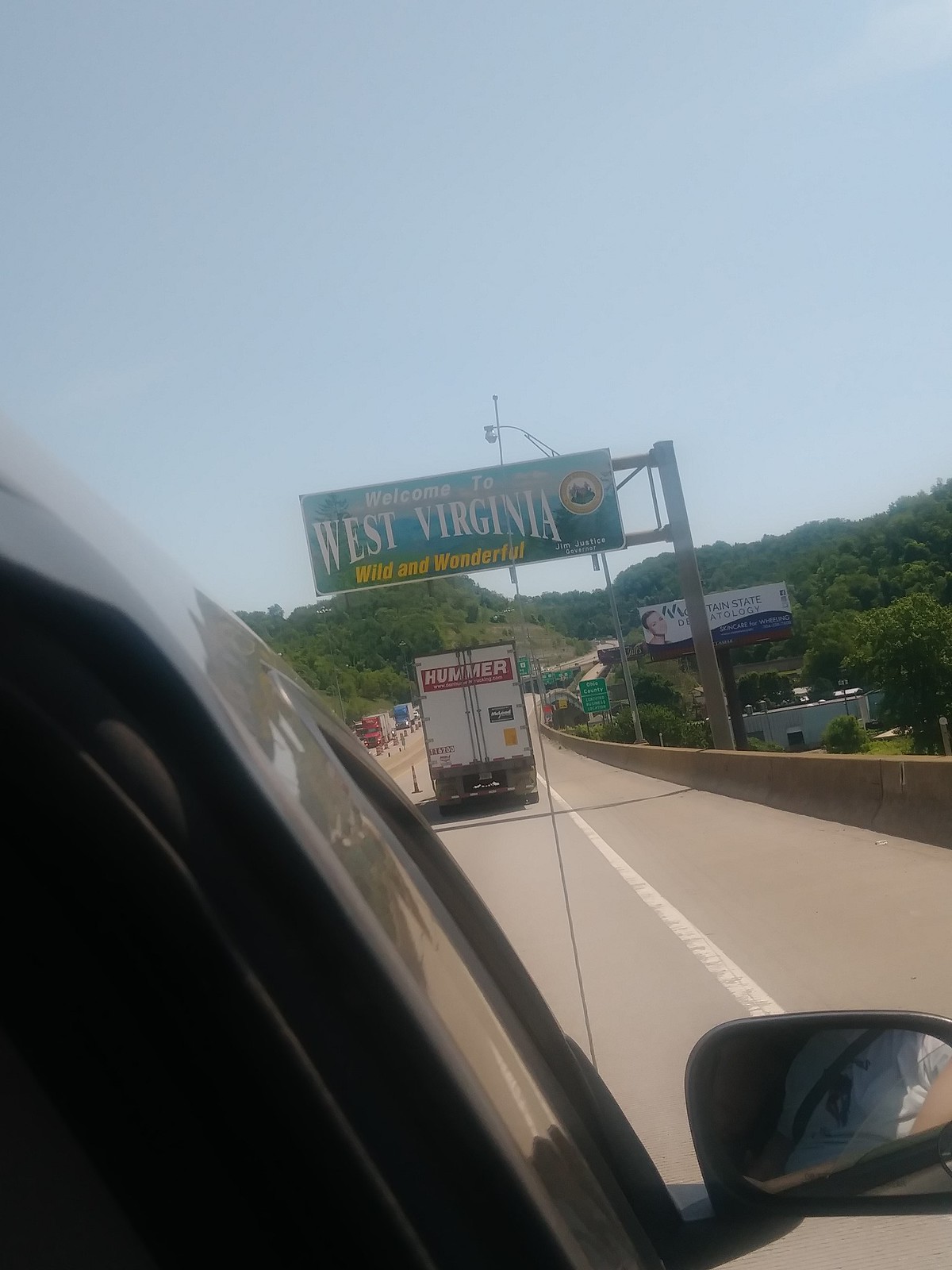Photographed from the passenger side of a vehicle, this image captures a vibrant moment on a highway entering West Virginia. In the foreground, the car's passenger side mirror is visible, adding depth to the scene. Dominating the center of the image is a prominent green "Welcome to West Virginia" sign, displaying a picturesque landscape of the state. The sign's white and yellow lettering reads, "Welcome to West Virginia" and "Wild and Wonderful," respectively. Ahead, a Hummer truck leads the vehicle from which the photo was taken, while several semi-trucks are visible on the opposite side of the median. Additional road signs and a billboard for dermatology services can be seen against a backdrop of lush, rolling trees under a clear blue sky.